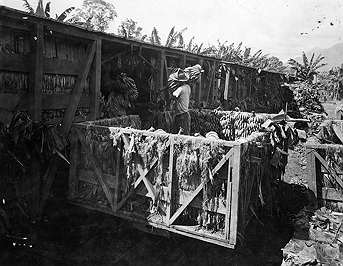The black and white photograph captures an old scene set in what appears to be a tropical banana plantation. The sky above is a mix of white and gray, adding a nostalgic atmosphere to the image. Central to the photo is a man wearing a round-brimmed hat, a white short-sleeved shirt, and work pants, carrying a large bunch of bananas over his shoulder. He is walking through a large wooden gate-like structure, which appears to be part of a deck or shelter. This structure leads into what looks like a storage area or train car, where other large bunches of bananas hang from hooks on the ceiling. Nearby, another person is seen walking towards the building with a batch of bananas, suggesting active collection and storage, perhaps for transportation. In the background, tropical trees, likely banana trees, add to the authenticity of the plantation setting. Scattered birds can be seen flying in the sky, enhancing the dynamic yet timeless quality of the scene.